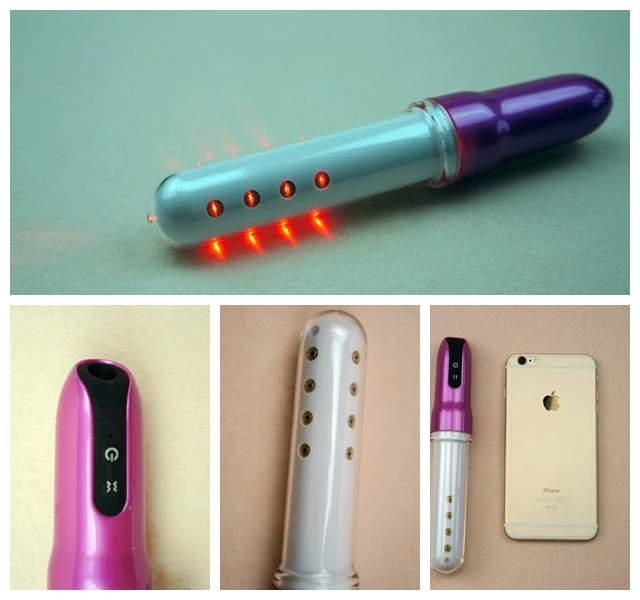This image is a detailed collage featuring four pictures of genotightening sticks against a green background. The top image, occupying half of the collage, showcases a cylindrical stick with a purple handle and a blue tip, which has four circular holes emitting lights. Below, three images are arranged side-by-side. 

In the bottom left image, we see a close-up of the handle, revealing a pin and a section with a black segment that has two buttons, one resembling a power symbol. The middle image zooms in on the tip of another similar stick, showing its white section with multiple holes arranged vertically. Finally, the bottom right image displays an iPhone placed face down, with its iconic Apple logo visible on the back. Next to it is another genotightening stick, this one featuring a purple handle and a white tip, providing a clear size comparison between the device and the phone.